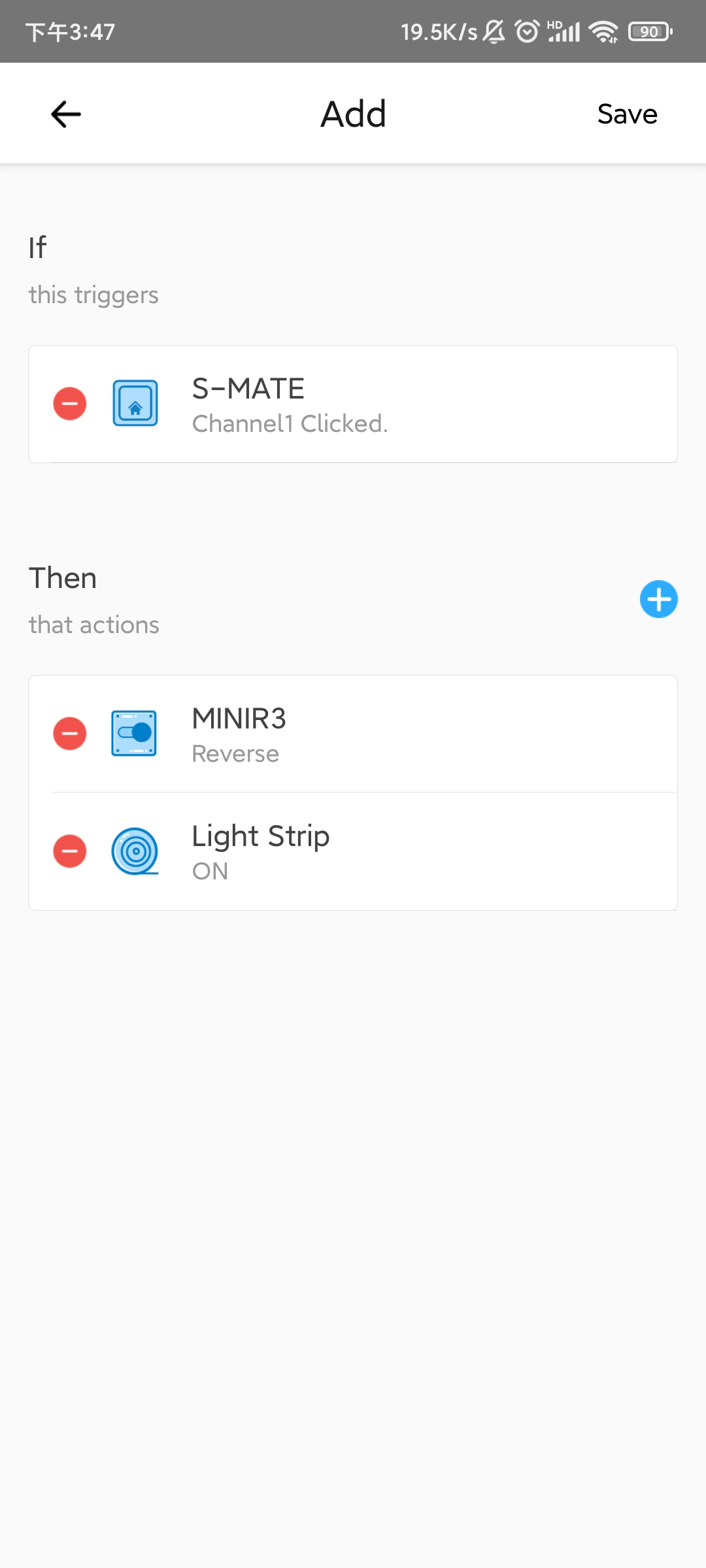Here is a detailed and cleaned-up caption for the given screenshot:

---

The screenshot of a smartphone screen shows a dark grey status bar at the top displaying the time as 3:47, a data rate of 19.5k/s, an alarm clock icon, full signal bars, full Wi-Fi signal, and an 80% battery level. Below the status bar, the screen has a white background featuring a black left arrow on the left side, the word "Add" centered, and the word "Save" on the right side. Underneath this, a section with a grey background reads "If This Triggers."

Below this heading, there's a white box containing a red circle with a line through it and a blue icon next to the text "s-mate, channel click." Following this, another section labeled "Then That Action" appears, featuring a blue circle with a plus sign in the middle. Beneath this, there are two options: "MINIR3 reverse" and "Light Strip On," each accompanied by a red circle with a line through it and a blue icon on the left side.

---

This caption provides a detailed and organized description of the various elements and their layout within the screenshot.